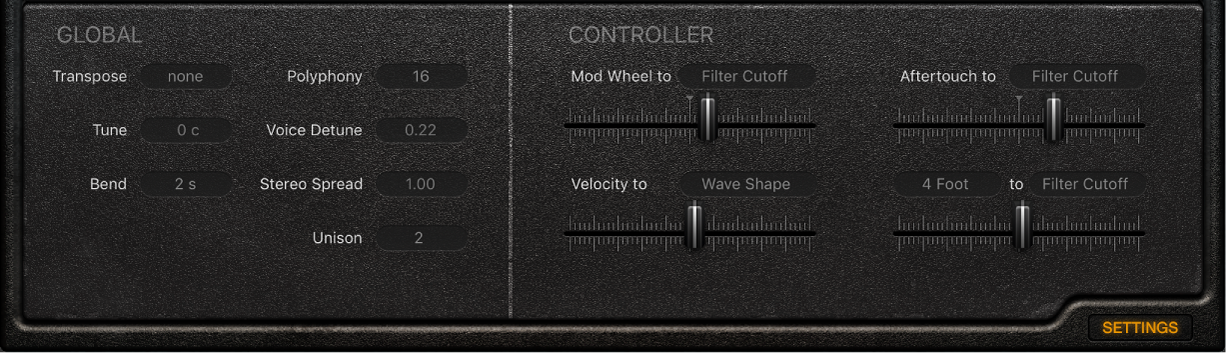This is a horizontally oriented photograph showcasing the front panel of a sophisticated black audio equipment controller. The surface is adorned with various controls and indicators. On the left-hand side, there's a section labeled "Global" at the top. This section includes adjustable settings for parameters such as transpose, tune, bend, polyphony, voice, detune, stereo spread, and unison. Each of these parameters has a corresponding digital window displaying numerical values.

On the right-hand side of the panel, the section labeled "Controller" features four slider knobs. These sliders are sequentially labeled as follows: "mod wheel to filter cutoff," "aftertouch to filter cutoff," "foot to filter cutoff," and "velocity to wave shape," allowing for detailed manipulation of the audio signal's characteristics. Each slider is accompanied by a descriptive label to indicate its function.

At the bottom right corner of the panel, the word "Settings" is elegantly embossed in gold, signifying the comprehensive nature of the controls available on this audio device. The various knobs, sliders, and digital readouts collectively suggest that this equipment is designed for detailed audio and music adjustments.